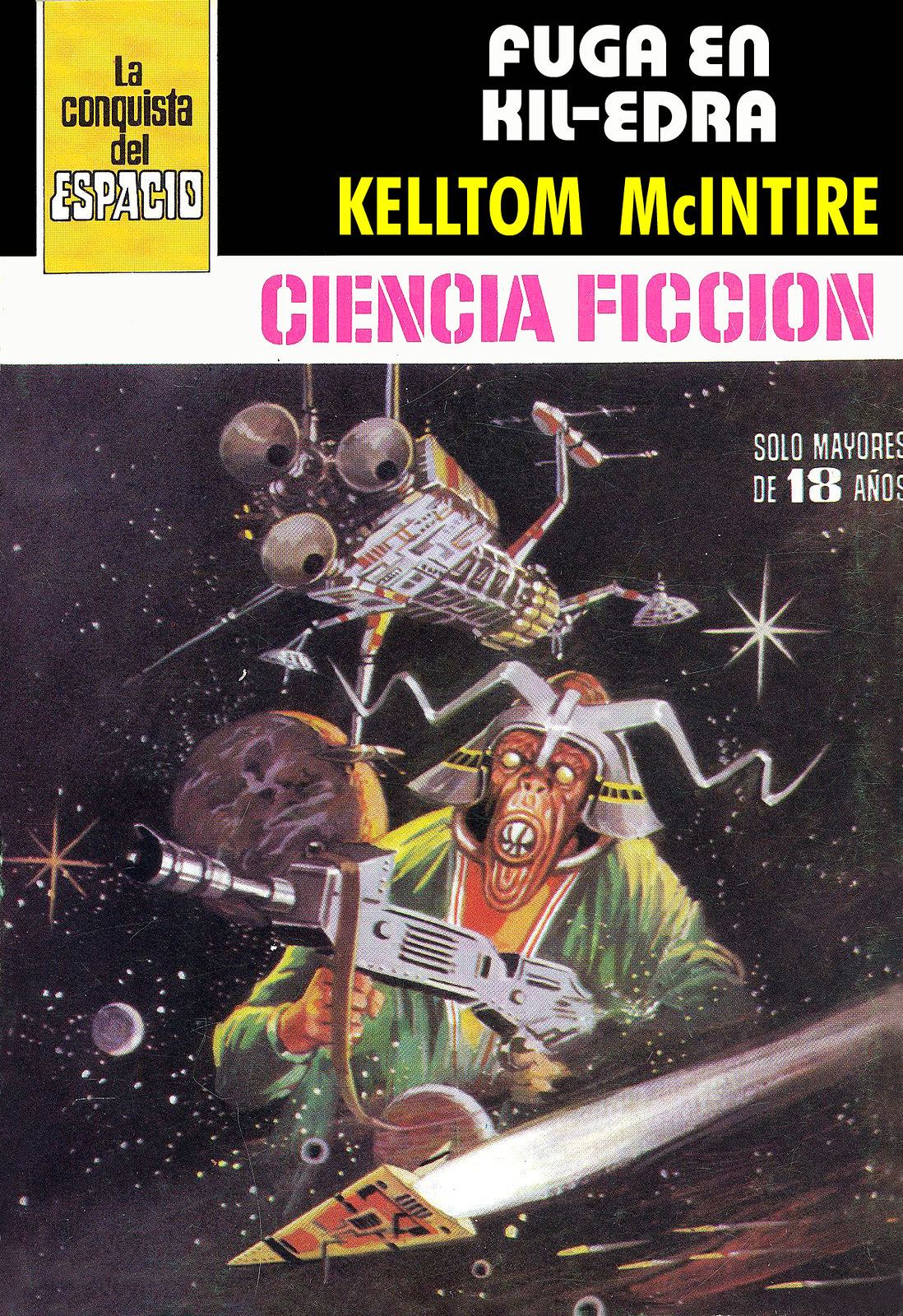The image appears to be an aged and faded comic book cover with a science fiction theme. At the top, there's a black border extending to the right. On the left side of this border, there's a yellow rectangular banner with black and white text that reads "La Conquista del Espacio." To the right of the banner, also on the black border, there are the white letters spelling "Fuga en Kil-Edra." Below these words, in yellow letters, is the name "Keltom McIntyre." 

Underneath the black border, a white section spans across with pink letters that spell "Ciencia Ficción." The main image depicts a cartoony, alien-like creature wearing a green coat and a samurai hat, holding a silver laser gun. Above the creature, there is a spaceship, and behind it, a planet is visible. The background is filled with stars on a black sky, providing a cosmic setting. Another spaceship appears below the planet, flying to the left, with more planets scattered in the background. The entire cover has a nostalgic, worn-out appearance, suggesting it might be from an old magazine or poster, and there is text in the top right corner that reads "Solo Mayores de 18 Años."